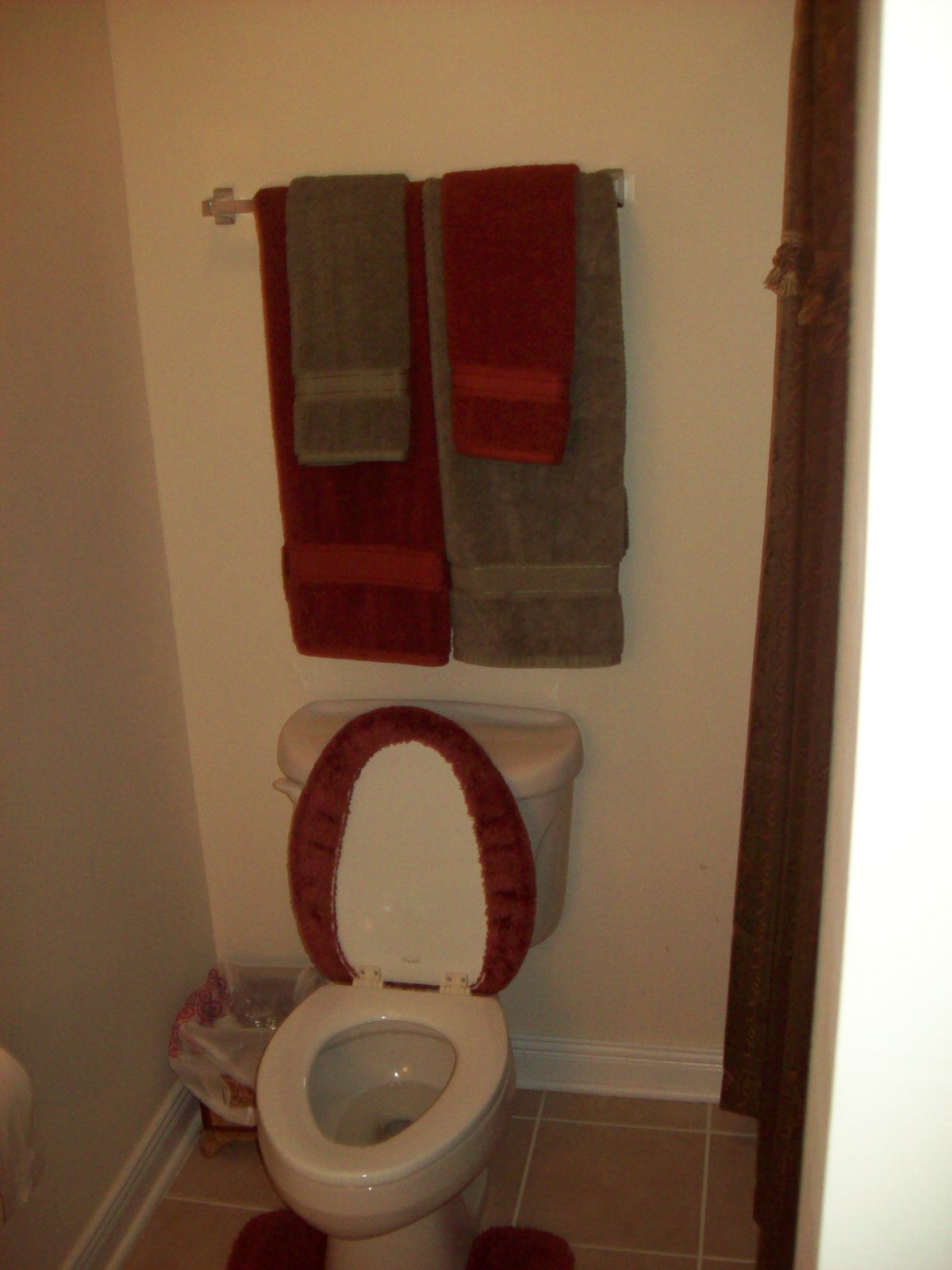This color photograph captures a detailed view of a 70s-style home bathroom, showcasing its unique decorative elements. The square tan-colored tile floor extends throughout the space, complementing the beige walls and white baseboard. Central to the image is an off-white, elongated oval toilet, with its lid up, revealing a plush deep burgundy red seat cover, which is echoed by a U-shaped rug at the base of the toilet. To the left of the toilet stands a trash can lined with a grocery bag, and just above the toilet paper dispenser peeks out from the bottom left corner.

Above the toilet, a stainless steel towel rack is mounted on the wall, adorned with a blend of towels. A large burgundy bath towel and a gray bath towel are hung with matching hand towels layered over them—gray over red on the left and red over gray on the right. Completing the room's decor, a brown curtain with fringe detail hangs to the side, possibly concealing a doorway. This detailed setup not only reflects the owner's taste but also enlivens the small space with a distinct retro vibe.